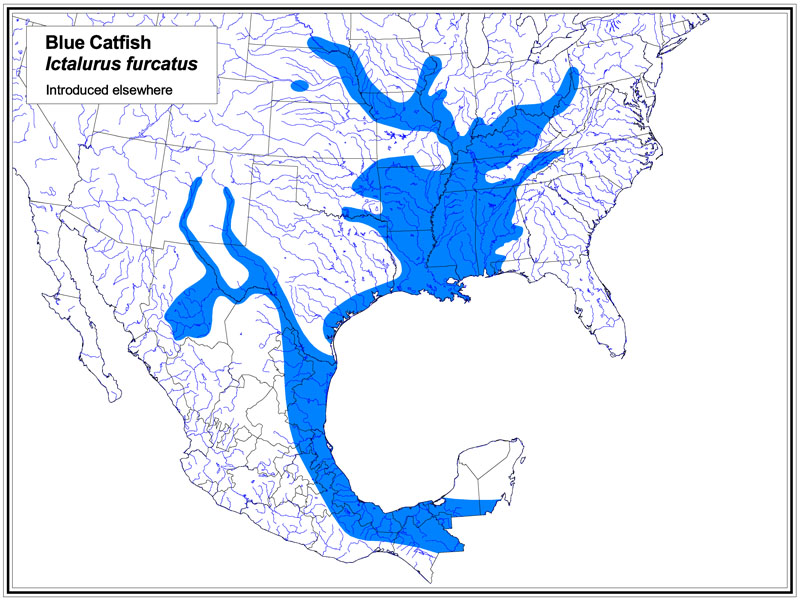The image depicts a map of the United States, characterized by a blue outline and white fill, with various splotches of light blue indicating specific locations. The background is white with a dark blue or black frame. In the upper left-hand corner, a small rectangle reads "Blue Catfish, Ictalurus furcatus, introduced elsewhere" in black text. The map highlights the distribution of the blue catfish, with blue areas particularly prevalent in parts of Alabama, Mississippi, Texas, Louisiana, and extending into Mexico. Notably, the depiction includes prominent blue markings near Florida, emphasizing the widespread introduction of the species in North America. The entire illustration is rendered in black, white, and shades of blue.